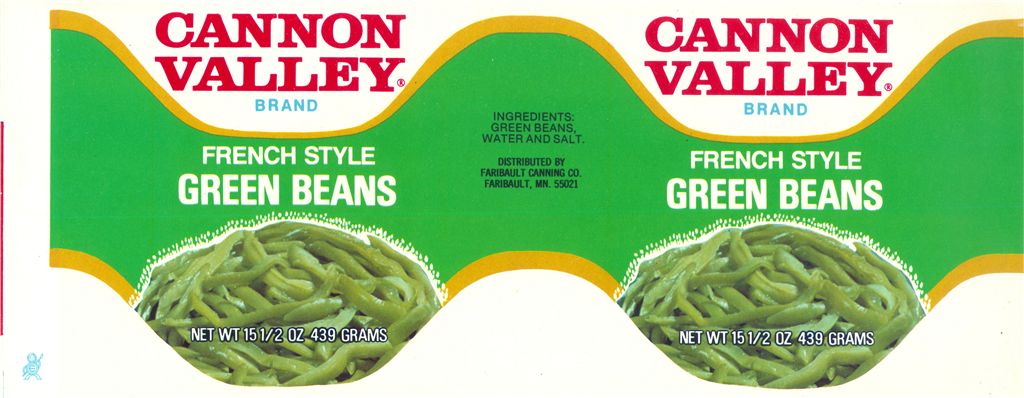The image showcases a label for Cannon Valley brand French-style green beans, repeated mirror-fashion to appear twice, side by side. The label features a white background with red "Cannon Valley" lettering and a blue "brand" underneath. A prominent green zigzag stripe, outlined in yellow, spans across the label and contains the text "French Style Green Beans" in large, white capital letters. Below the text, there's an image of cooked green beans, accompanied by the white text "Net Wt 15.5 oz (439 grams)." The central green band also lists ingredients as "green beans, water, and salt" and indicates that the product is distributed by Faribault Canning Company, Faribault, MN 55021. The right side of the label is an identical copy of the left, as the entire label is designed to wrap around a can.